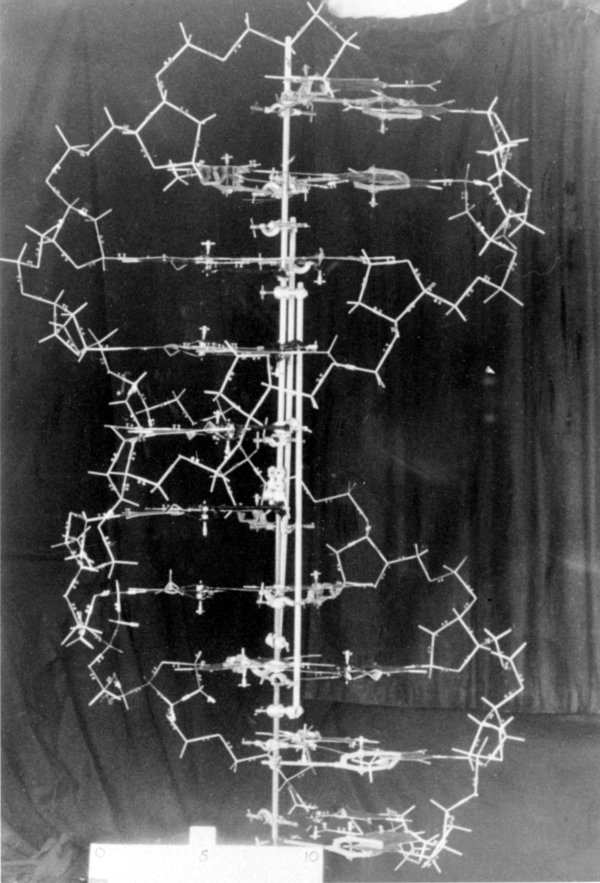This grainy, vintage black-and-white photograph, likely taken 50 or 60 years ago, showcases a mysterious 3D model situated against a textured gray curtain backdrop. The central model features interconnected branches, some forming partial hexagon shapes, supported by three vertical poles. Spiral wires encircle these branches, reminiscent of a DNA molecule or double helix structure, possibly indicating a scientific exhibit related to DNA or chemistry. Additionally, there appears to be a small figurine nestled within the branches and a ruler marked with the numbers 0, 5, and 10 at the base, further suggesting the model's scientific purpose. Despite the low-quality image, the intricate details and sharp wire extensions accentuate its complexity and potential educational significance.